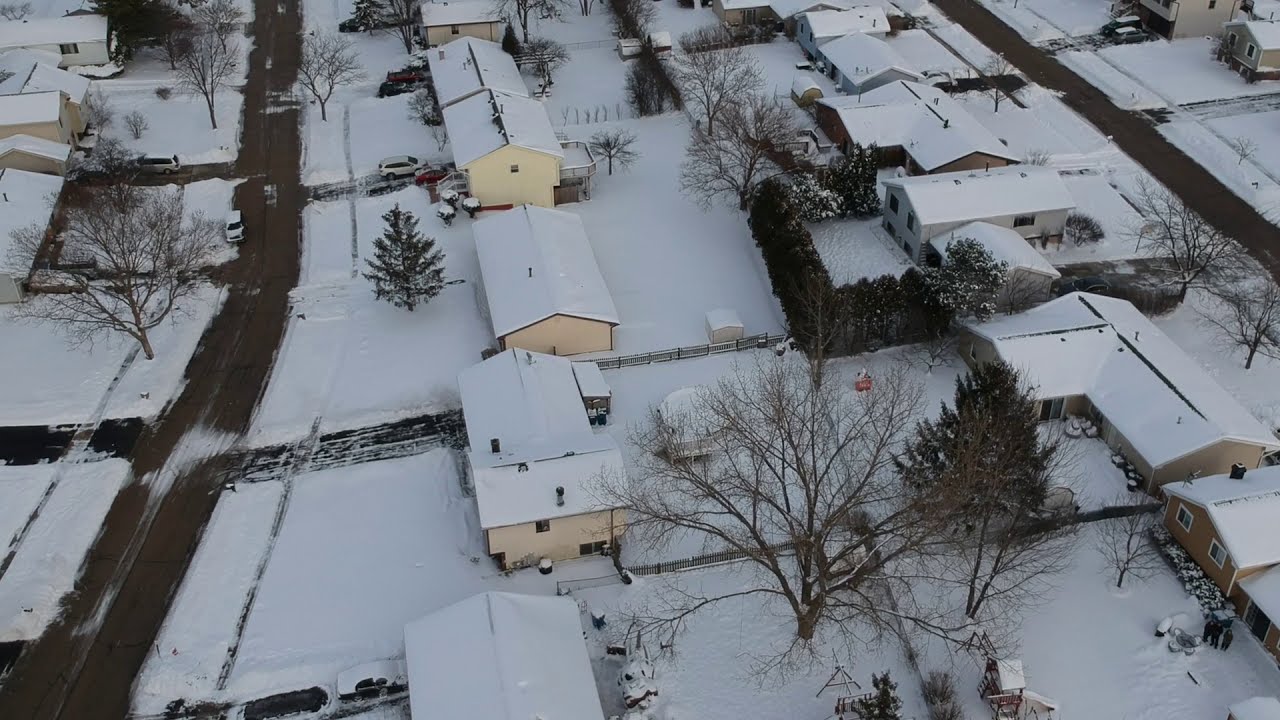This image presents an aerial view of a peaceful residential neighborhood blanketed in winter snow. The scene is framed vertically, with distinct rows of houses on the left and right sides, creating a symmetrical layout. Snow covers the ground, rooftops, and bare tree branches, adding a serene, white hue to the landscape. Interspersed among the snow-covered trees, you can spot resilient green pine trees. 

The roads, which run along the far right and left sides of the image, contrast the snowy backdrop with their dark brown or black surfaces, occasionally dotted with icy patches. Various cars are visible, parked in driveways and along the streets, with colors ranging from red, white, and tan to cream and black. Notably, a white van and a white SUV are distinguishable in the scene, their roofs partially hidden under a layer of snow.

At the center of the image, backyards filled with trees extend vertically, creating a natural divider between the two rows of houses. The combination of snow-covered landscapes, seasonal trees, and residential structures encapsulates the quiet and stillness of a neighborhood in winter.